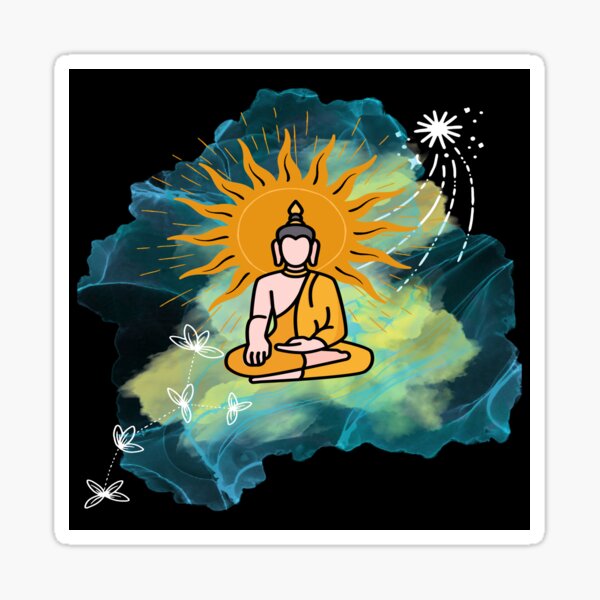The image showcases a digital art piece of a faceless figure, resembling a monk or a meditating individual, positioned centrally in a lotus pose. The figure is wearing an orange, long-sleeved onesie with the right shoulder exposed. They are barefoot and bare-handed, with a small ponytail embellished with gold at the top of their head, accompanied by a gold necklace. Surrounding the head is an encompassing sun with a small yellow ring at its center, predominantly orange with small black lines along the rays. Behind the figure, the background is filled with vibrant blue and yellow splotches, complemented by hints of green and orange. A white border frames the black backdrop of the image. Decorative elements include a drawn star in the upper right-hand corner and interconnected white flowers with dotted lines in the bottom left-hand corner.